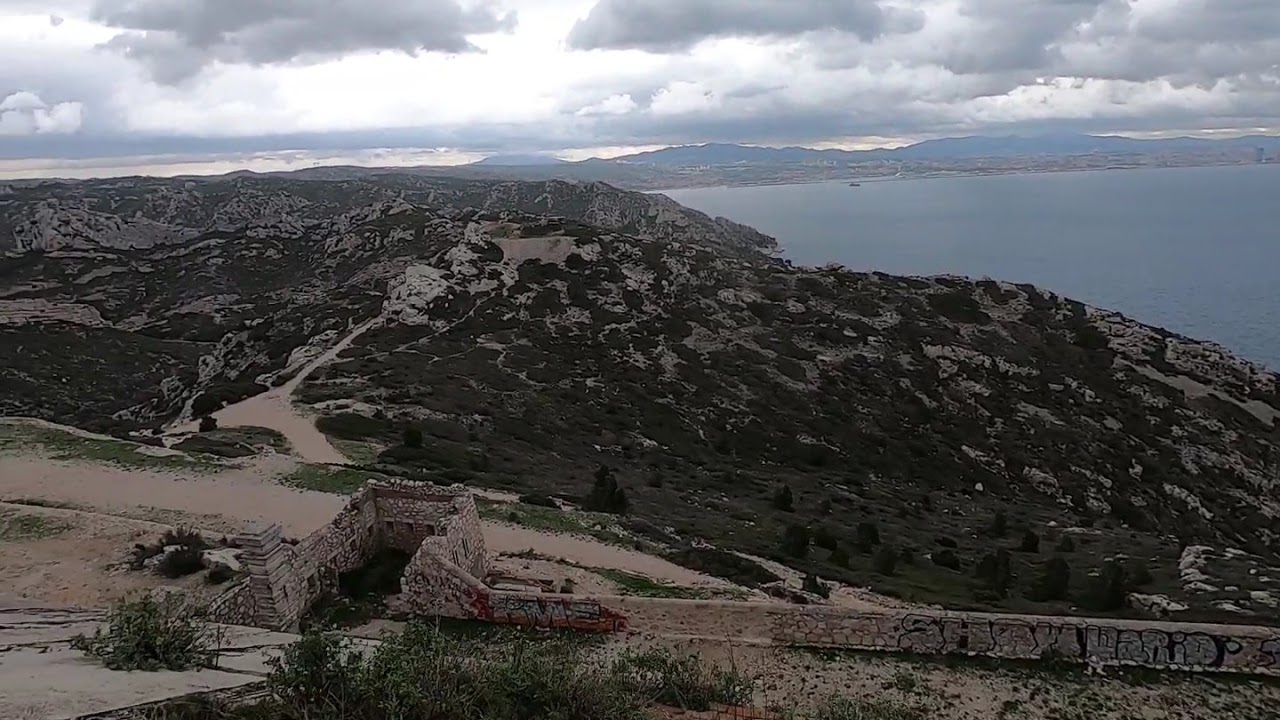The aerial view captures a sprawling hilly landscape dominated by the ruins of an ancient stone wall in the forefront, which is partially crumbling and adorned with various graffiti. The bottom left of the image features a cement-like slope leading up to this wall, while a flat, tan-colored dirt road stretches in front of it. This road continues into the distance, weaving through verdant hills speckled with occasional brown and white bare patches. Further out, a vast, calm, blue body of water contrasts sharply with the lush greens of the hills. Even farther back, majestic mountains rise under a heavy gray sky, thick with clouds that cast shadows over the landscape, enhancing the texture and depth of this outdoor scene.